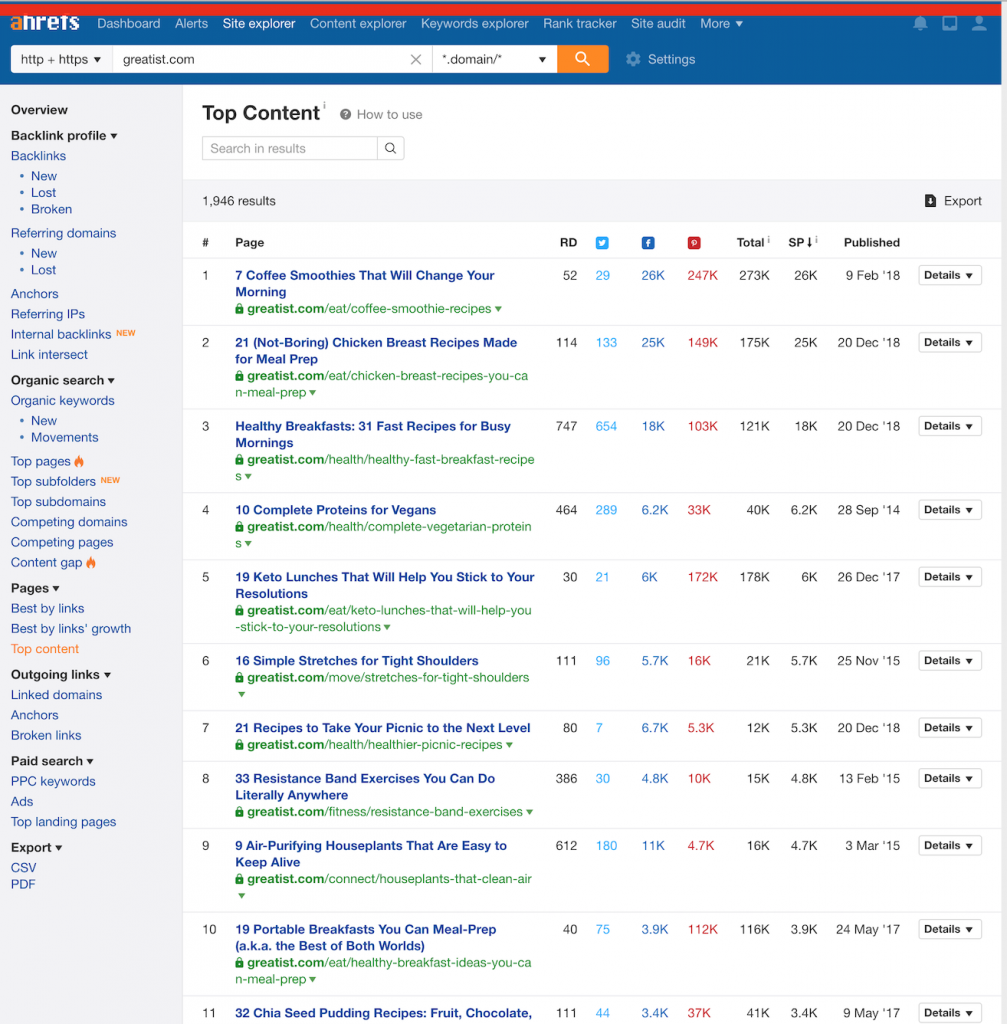The screenshot displays the interface of a sophisticated SEO tool on a website likely named "greatlist.com" or "greatest.com." At the very top, there is a red navigation bar featuring options such as 'Dashboard,' 'Alerts,' 'Site Explorer,' 'Content Explorer,' 'Keywords Explorer,' 'Rank Tracker,' 'Site Audit,' and more, alongside an HTTPS secured site indicator.

On the left side, a detailed sidebar lists various analytical categories including 'Overview,' 'Backlink Profile,' 'New,' 'Lost,' 'Broken Links,' 'Referring Domains,' 'Anchors,' 'Referring IPs,' 'Internal Backlinks,' 'Link Website,' 'Query and Search,' 'Find Keywords,' 'New Movements,' 'Top Pages,' 'Top Subfolders,' 'Top Subdomains,' 'Competing Domains,' 'Competing Pages,' 'Content Cap,' 'Pages Best by Links,' 'Best by Links Growth,' 'Echo and Links,' 'Link Domains,' 'Anchors,' 'Book Links,' 'Page Search,' 'PPC,' 'Keywords,' 'Ads,' 'Top Line Pages,' and options for export in CSF or PDF format.

The main content of the interface highlights various articles and resources such as "Seven Coffee Smoothies to Transform Your Morning," "21 Not-Boring Chicken Breast Recipes for Meal Prep," "Healthy Breakfasts for Super Busy Mornings," "Technically Potent Vegan Options," "33 Resistance Band Exercises You Can Do Anywhere," "9 Easy-to-keep-alive Houseplants," "Portable Breakfast Ideas for Meal Prep," and "32 Pudding Recipes including Fruit and Chocolate." These headings suggest a blend of lifestyle, fitness, and culinary content aimed at readers seeking practical advice and ideas.